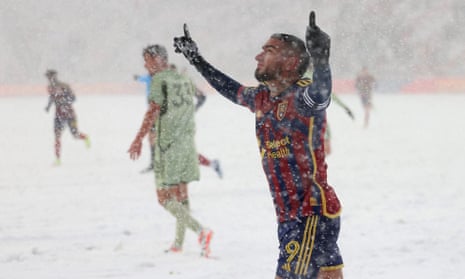In this detailed photograph capturing an unusual scene of a soccer game played amidst heavy snowfall, the visibility is significantly obscured by the large snowflakes descending from the sky, and the thick layer of snow blanketing the ground. The foreground prominently features a soccer player, possibly of Indian or Hispanic descent, raising both arms with a finger pointing skyward from each hand, giving an impression of triumph or signaling “number one”. He is adorned in a dark red and navy striped shirt, paired with dark blue shorts accentuated by yellow stripes and the number nine. His facial features include a small beard or goatee. Surrounding him, albeit more indistinctly due to the swirling snow, are other players. One close behind is dressed in a light green uniform, while others in red and navy can be seen further back, their figures blurred by the wintry conditions. The backdrop of the snowy field is framed by a red wall, faintly visible through the dense snowfall.